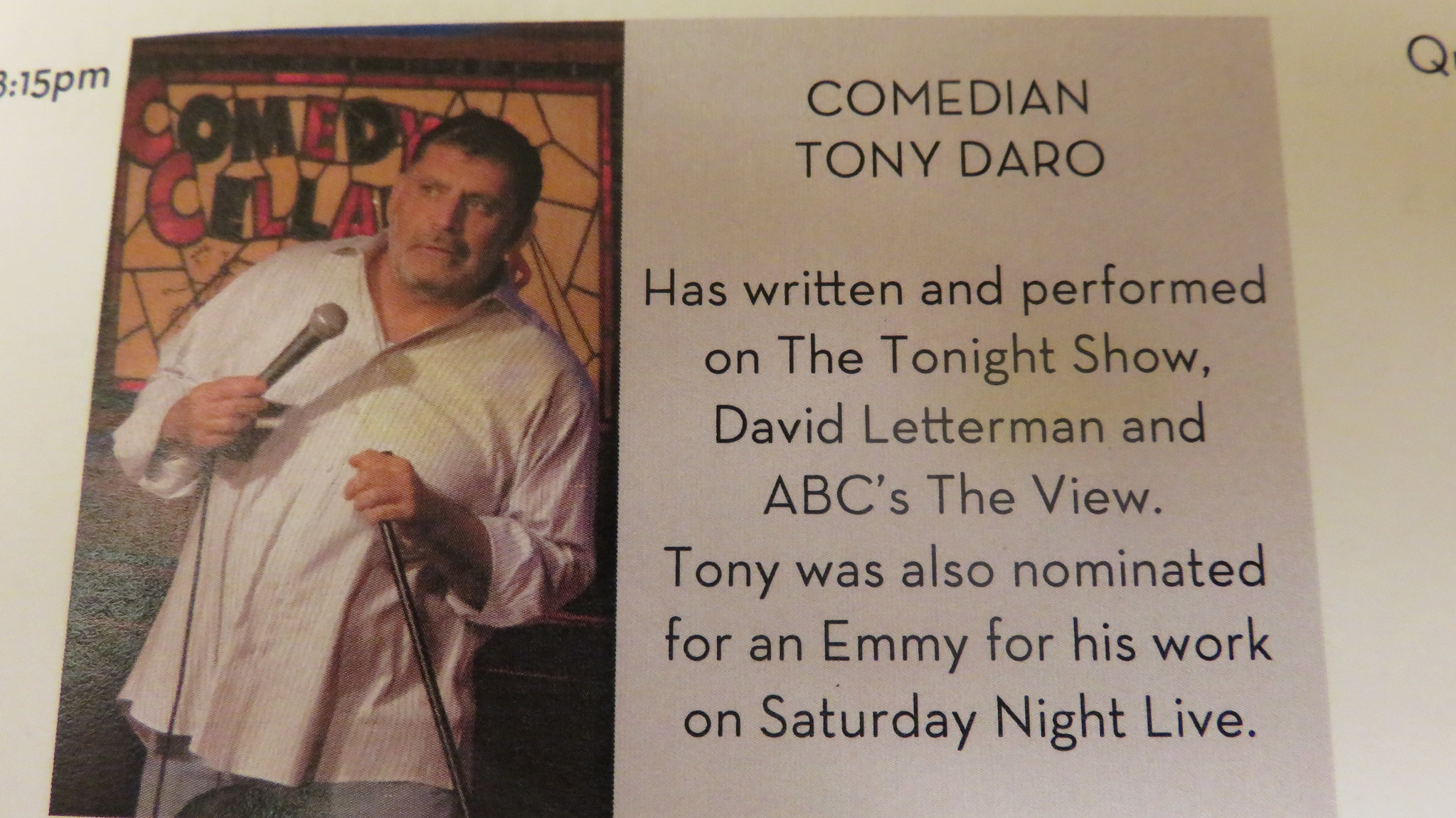In the image, on the left-hand side, there is a photograph of a man named Tony Darrow, a comedian with short dark hair and a lightly unshaven face, sprinkled with gray. He is wearing a white, untucked collared shirt that has a subtle mix of white and red, fully buttoned down, paired with blue jeans. Tony is holding a black microphone in his right hand while resting his left hand on the black microphone stand. Behind him, a yellow, red, and green stained-glass window prominently features the sign "Comedy Cellar," although part of the letters "Y" and "R" are obscured by his head. A wired microphone cord extends from the center-left to the bottom-left of the image. To the right of the photograph is a light gray background containing a detailed biography in black lettering. It reads: "Comedian Tony Darrow has written and performed on The Tonight Show, David Letterman, and ABC's The View. Tony was also nominated for an Emmy for his work on Saturday Night Live." The overall setup and layout suggest this image is part of a magazine or program page.